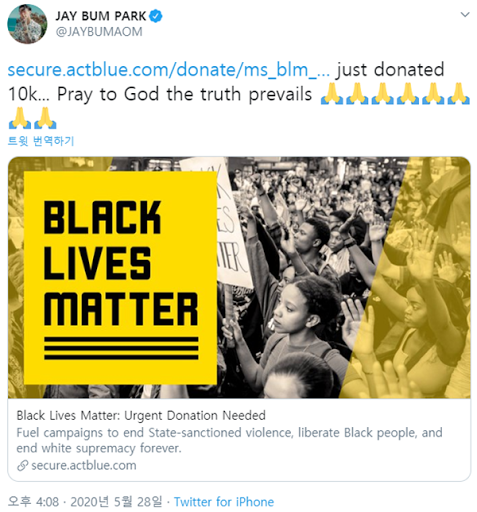The image features a verified Twitter account belonging to an individual named J Bomb Park. The blue checkmark next to the username signifies the account's verified status. Beneath the username, a blue hyperlink directs users to a donation page at secure.actblue.com. The tweet indicates a donation of $10,000 with a message praying for the truth to prevail, accompanied by multiple praying hands emojis.

In Japanese text, the tweet mentions Black Lives Matter and introduces a banner with a yellow background and black text stating "Black Lives Matter" across three lines. It appeals for urgent donations to support campaigns aimed at ending state-sanctioned violence. The same donation link appears again below this text.

The tweet is noted as being posted via Twitter for iPhone. To the right of the yellow banner, there is an image showing a group of people with their hands raised in protest. Among them is a young woman, likely in her mid-20s, holding a sign that reads "Black Lives Matter." The crowd, primarily composed of Black individuals, is actively engaging in the protest, underscoring the movement's call for equality and justice.

This tweet serves both as an informational post about the Black Lives Matter movement and a call to action for donations.